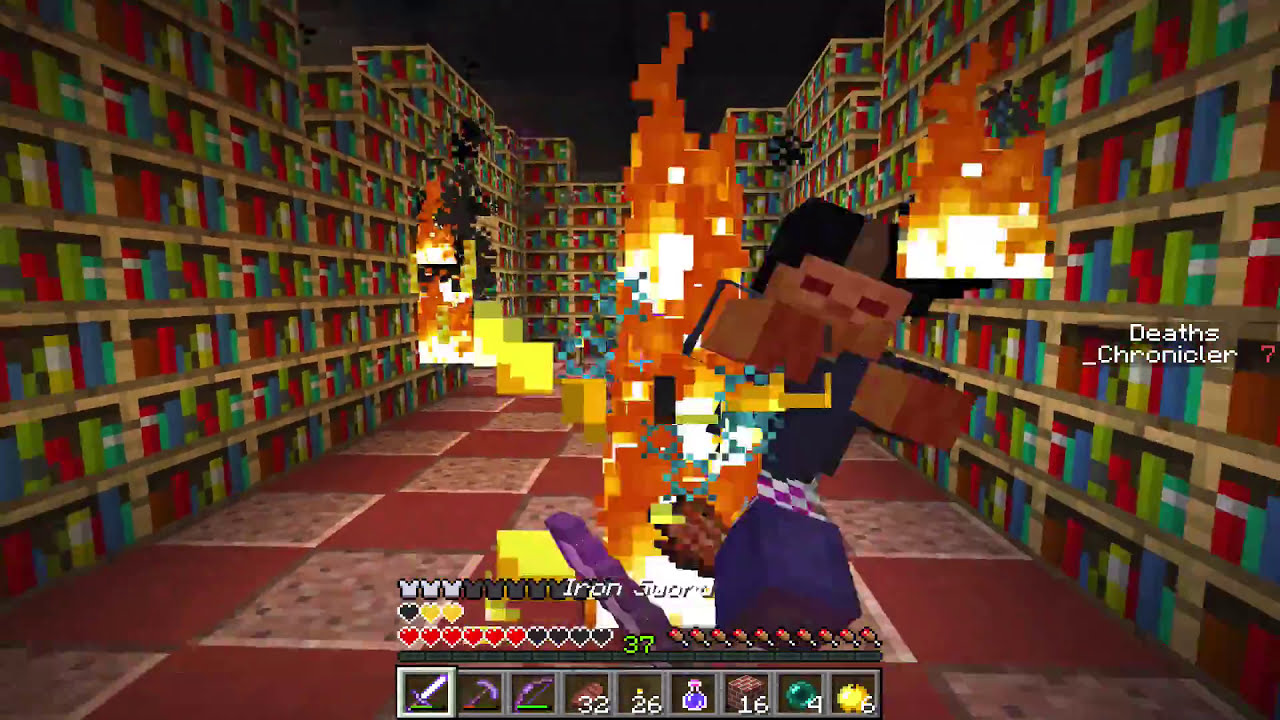This image portrays a detailed video game scene from Minecraft, showing a character in a perilous situation. The horizontally rectangular screen displays an interior library setting, lined with towering bookshelves filled with multicolored books on both the left and right sides, creating a sense of depth. The floor is checkered with red tiles, contributing to the library's structured appearance.

In the foreground stands a blocky Minecraft character with dark hair, dressed in a blue shirt and bottoms. The character appears to be running towards the player, engulfed in flames, with a mix of yellow, orange, and white blocks depicting the fire behind him. To the right of the character, white text reads "Death's Chronicler?" suggesting a possible in-game character or event. The character appears to be mid-fall, adding to the visual intensity of the scene.

Along the bottom of the screen is the UI displaying the character's stats and inventory. The health bar shows a mix of colors indicating the player's current status: 2 yellow hearts and 6 red hearts out of 10, along with a few black ones. The armor bar above the health shows the player has 3 defense points left. The inventory section includes icons for an iron sword, pickaxe, bow and arrow, and various items like meat, yellow items, a purple bottle, 16 bricks, 4 green orbs, and 6 yellow fruits. The presence of these items suggests the character's preparedness for the challenges at hand, despite the current threat of fire.